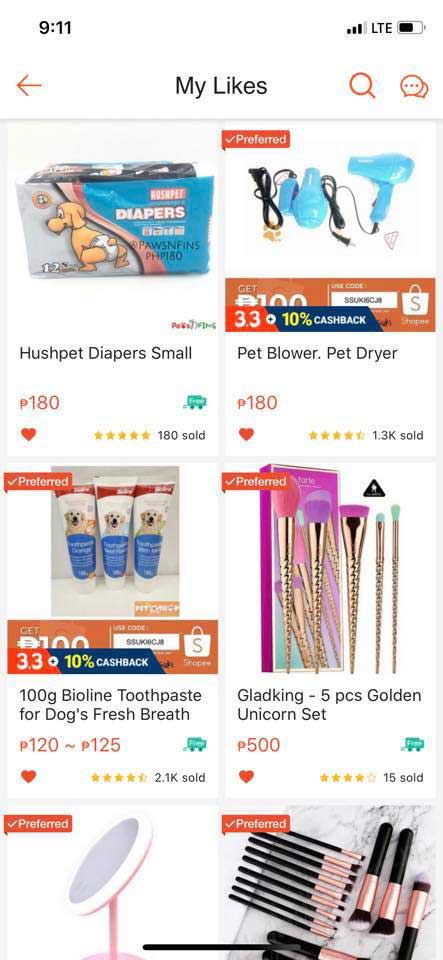In the image, there is a section titled "My Likes" at the top, with black text displaying the user's preferred products. The interface includes an orange search icon and comment button in the top right corner, alongside an orange back button in the top left.

The image showcases six products favored by the user, all marked with a red heart to indicate their liked status:

1. **Top Left**: "Hushpest Deadpast Smudge P180" is a blue and gray pet product featuring a brown dog wearing a diaper. It has a 5-star rating in yellow, and has sold 180 units.

2. **Top Right**: "Pet Blower Pet Dryer" priced at 180, is a blue blower with a black coat and a "Preferred" sticker. It holds a rating of 4. something stars and has sold 1.3k units.

3. **Center Left**: This is a 100-gram "By Lining Toothpaste for Dogs" aimed at giving fresh breath, priced between 120 to 125. The product is rated 4.5 stars and has sold 2.1k units. The image depicts three packages featuring pictures of a brown dog, with blue, white, and red colors.

4. **Center Right**: "Glad King Five Pieces Golden Unicorn Set" costs 500 and is gold in color, with a 4-star rating and 15 units sold.

5. **Bottom Left and Bottom Right**: Two additional products are displayed at the bottom of the image, though details about these products are not provided in the description.